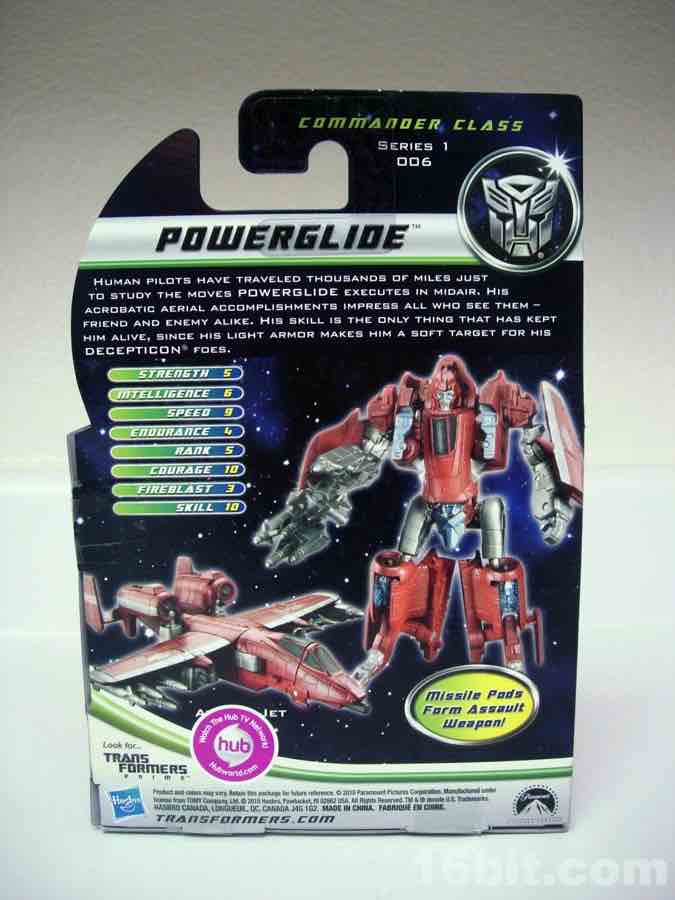This detailed caption encapsulates the provided descriptions:

The image is the back of a Transformers toy box, predominantly black with a space-themed background featuring stars. At the top, it displays the text "Commander Class Series 1026." In the top right corner, there is an icon: a silver mask set within a circle. Below this, the name "Power Glide" is prominently displayed. Accompanying this name is a descriptive paragraph: "Human pilots have traveled thousands of miles just to study the moves Power Glide executes in mid-air. His acrobatic aerial accomplishments impress all who see him, friends and enemy alike. His skill is the only thing that has kept him alive since his light armor makes him a soft target for his Decepticon force." Below this paragraph are Power Glide's rankings: strength 5, intelligence 6, speed 9, courage 4, rank 5, fireblast 3, skill 10. The toy’s two forms are depicted: to the left, the red and silver jet, and to the right, a red and silver robot with red body and head, silver arms, and silver thighs. Further details about the product are noted at the bottom, including references to the makers Hasbro and TOEI, the official Transformers website, and additional product details in white and black text.